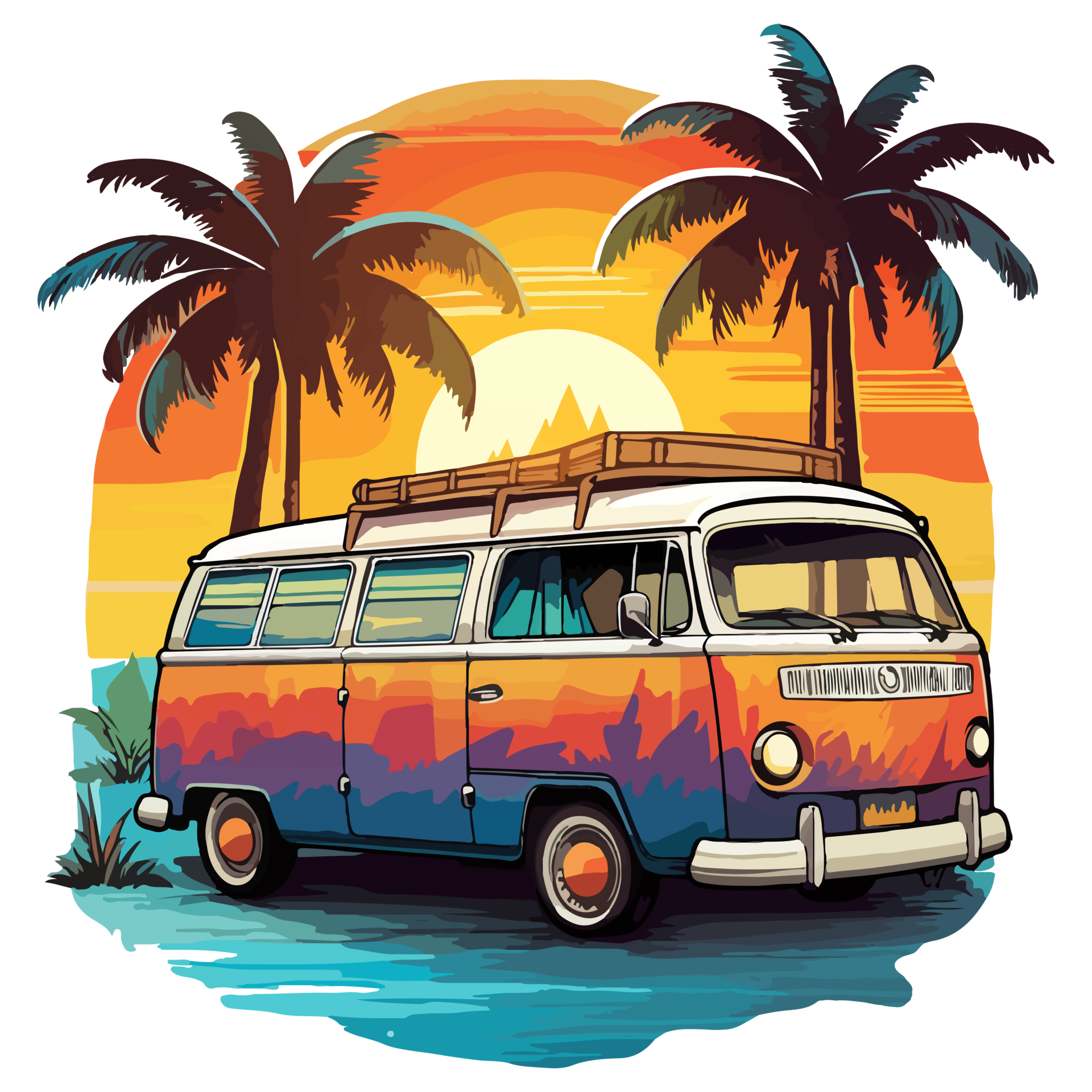The image is a vibrant and artistic depiction of a classic VW camper van, illustrated with a combination of digital and watercolor techniques. The van is parked centrally under two tall palm trees, their fronds gracefully arching downward. The camper van stands out with its striking color gradient, starting with a darker blue at the rough-textured bottom, which might represent a landscape silhouette. This blue transitions into layers of purple, red, orange, and lighter orange, and culminates in yellow towards the window section. The van's top is white and features a brown luggage rack mounted on it.

The scene behind the van is equally captivating, showcasing a dramatic sunset with hues of orange, yellow, and red. Sharp, shadowy mountains appear beneath the vibrant sky, adding depth to the composition. The ground on which the van is parked is painted in a blue tone, complementing the overall color scheme. Despite the detailed and colorful presentation, the van lacks any identifying plates or markings, enhancing its universal and timeless appeal. The wheels of the van are notably orange, and there are three rear windows plus the usual side windows and windshield in the cab.

In the foreground, hints of greenery or shrubbery add texture to the landscape, blending seamlessly with the artistic theme of camper life depicted in this picturesque scene. The entire composition paints a lively, dreamy, and nostalgic image of a vacation spot, capturing the essence of a carefree journey under a tropical sunset.